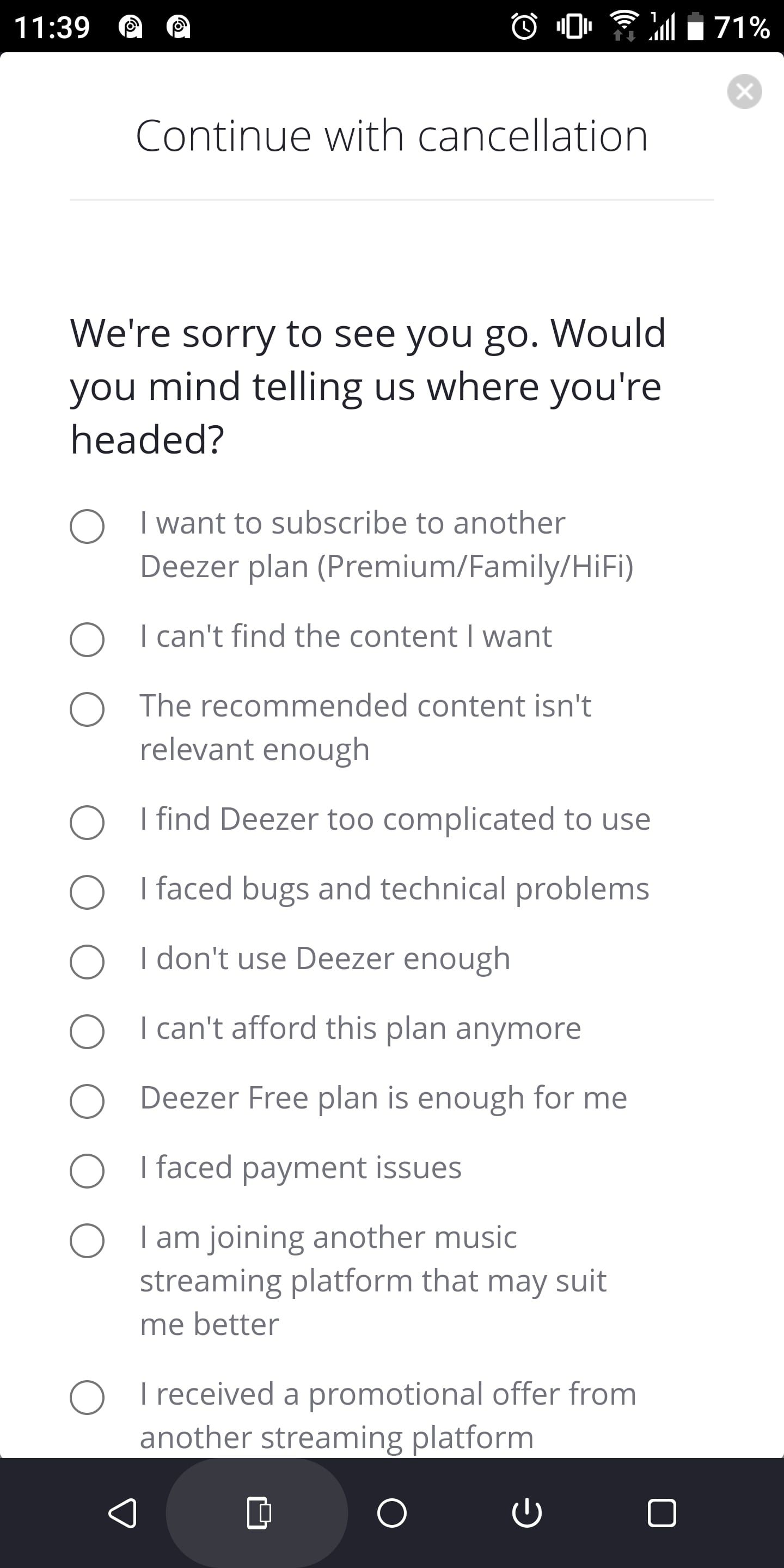The screenshot depicts a cancellation confirmation notice for the Deezer music streaming service. At the top of the screen, the option "Continue with cancellation" is clearly visible. Below this, a message expresses regret: "We're sorry to see you go. Would you mind telling us where you're headed?" This is followed by a series of selectable buttons arranged in rows, each providing a different reason for cancellation.

1. "I want to subscribe to another Deezer plan, either Premium, Family, or HiFi."
2. "I can't find the content I want."
3. "The recommended content isn't relevant enough."
4. "I find Deezer too complicated to use."
5. "I faced bugs and technical problems."
6. "I don't use Deezer enough."
7. "I can't afford this plan anymore."
8. "Deezer Free plan is enough for me."
9. "I faced payment issues."
10. "I am joining another music streaming platform that may suit me better."
11. "I received a promotional offer from another streaming platform."

None of these options have been selected by the user. The user appears to be in the process of interacting with one of the buttons on the bottom of the phone's interface. These bottom navigation buttons, displayed on a navy blue background, include (from left to right): a play button, a general home button, a power button, and a stop button.

The image captures these details on a mobile phone screen, offering a comprehensive view of the cancellation process and available options for users considering leaving the Deezer service.